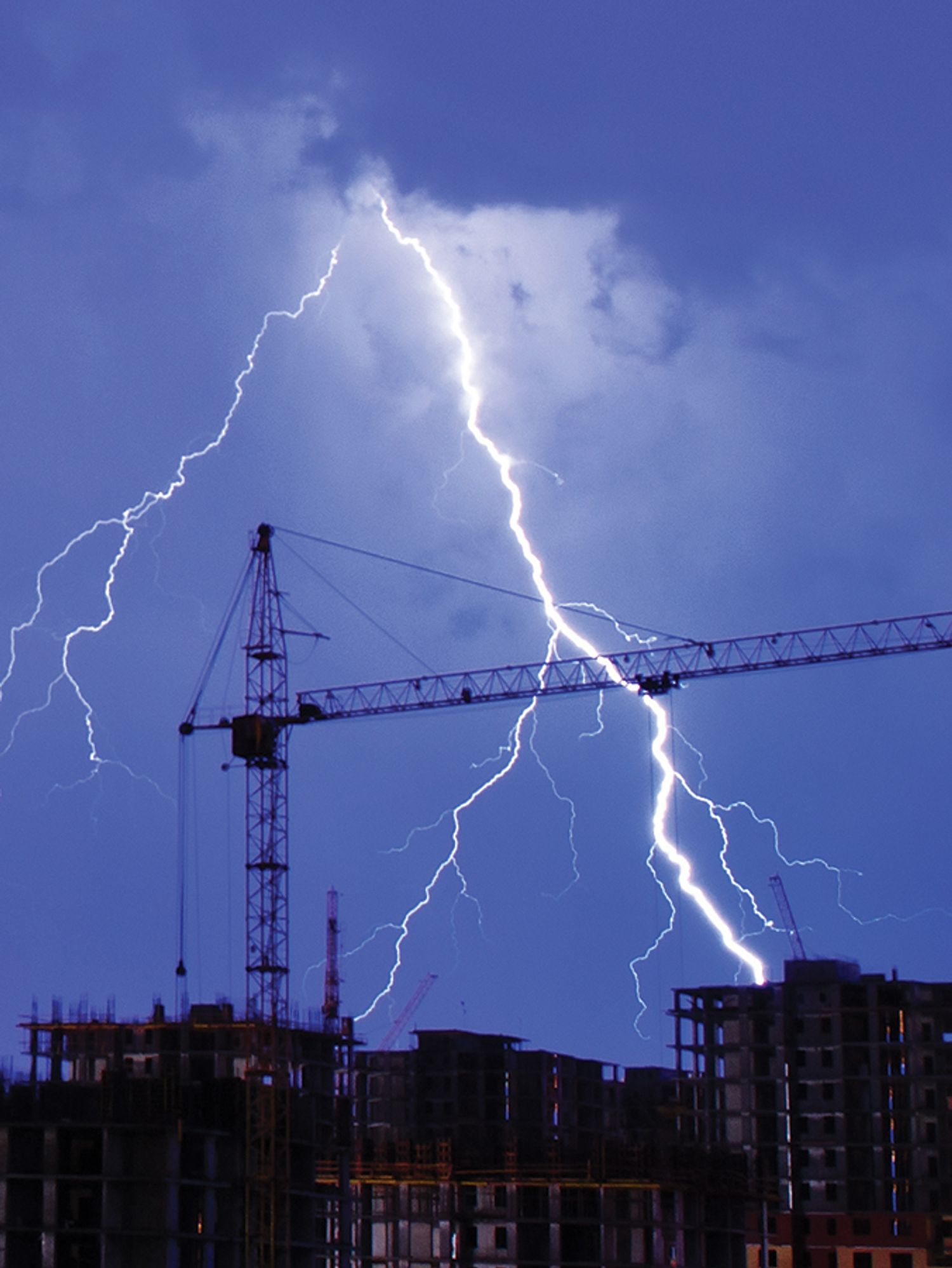This is a long exposure photograph of a city at night, capturing a dramatic scene of a lightning bolt striking amidst a dark, stormy sky. The rectangular image shows a night sky that takes up about three-fourths of the frame, filled with thick gray clouds appearing illuminated where the lightning bolt breaks through. The bolt, which splits into two branches, highlights the ominous night with its blinding brightness, making the clouds appear whiter in the center. Below the turbulent sky, a large construction site dominates the foreground, featuring multiple high-rise buildings in progress. These towering structures, which may eventually become apartments, have visible metal scaffolding and are framed by a massive construction crane extending about 10 stories high. The lower floors of the buildings are painted yellow, while the upper parts remain shadowed, the intricate details of their ongoing construction silhouetted against the striking display of nature’s power.